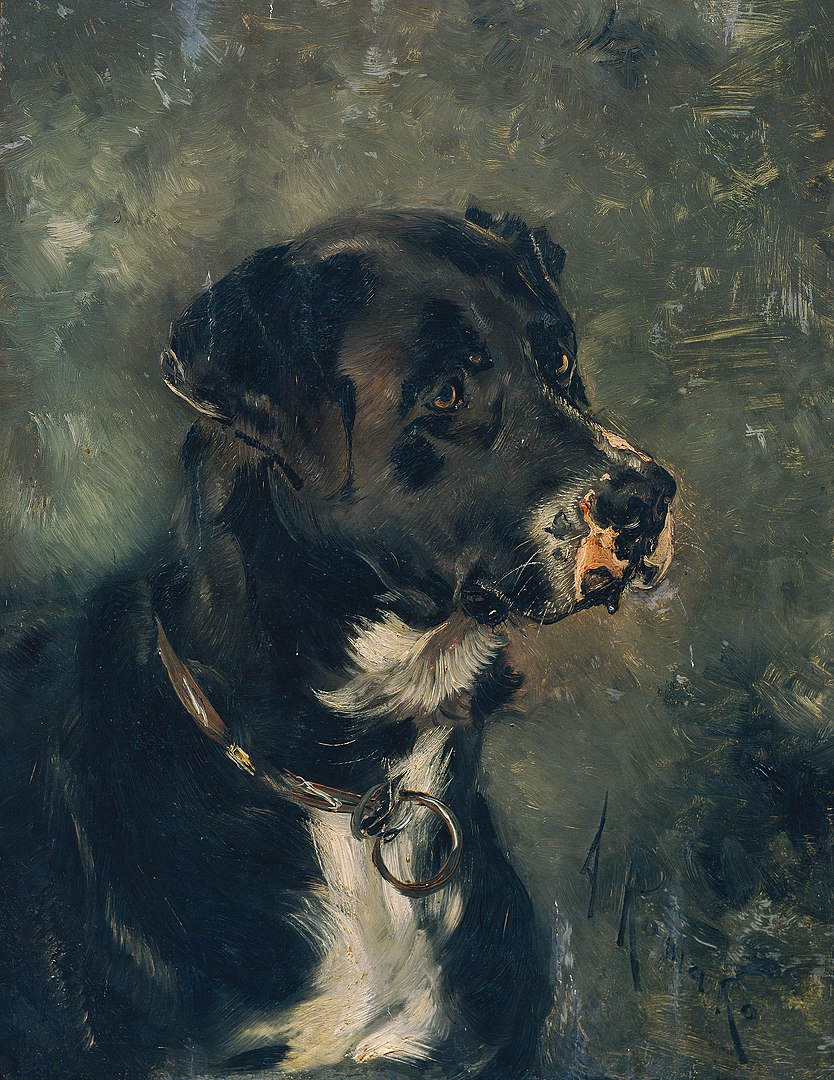This painting, titled "Head of a Butcher's Dog" by Anton Romako, is a skillfully crafted oil portrait in a somewhat realistic style, created around 1880. The large black dog, who occupies most of the canvas, has a pronounced white chest and some tan around his snout, with pinkish flesh visible at the tip of his nose. His eyes are a distinct yellowish-brown, contributing to his serious and somber expression. The dog wears a brown collar featuring a silver ring attachment, emphasizing his readiness for a leash. The background employs an impressionistic stroke effect of olive green, brown, and muted neutral colors, enhancing the painting's melancholic tone. The overall aesthetic, while not hyper-realistic, renders the dog lifelike, blending into a backdrop of mostly dark, neutral hues, with occasional splashes of brighter brown and yellow. The detailed yet somber portrayal is accentuated by the absence of any visible text in the artwork itself.